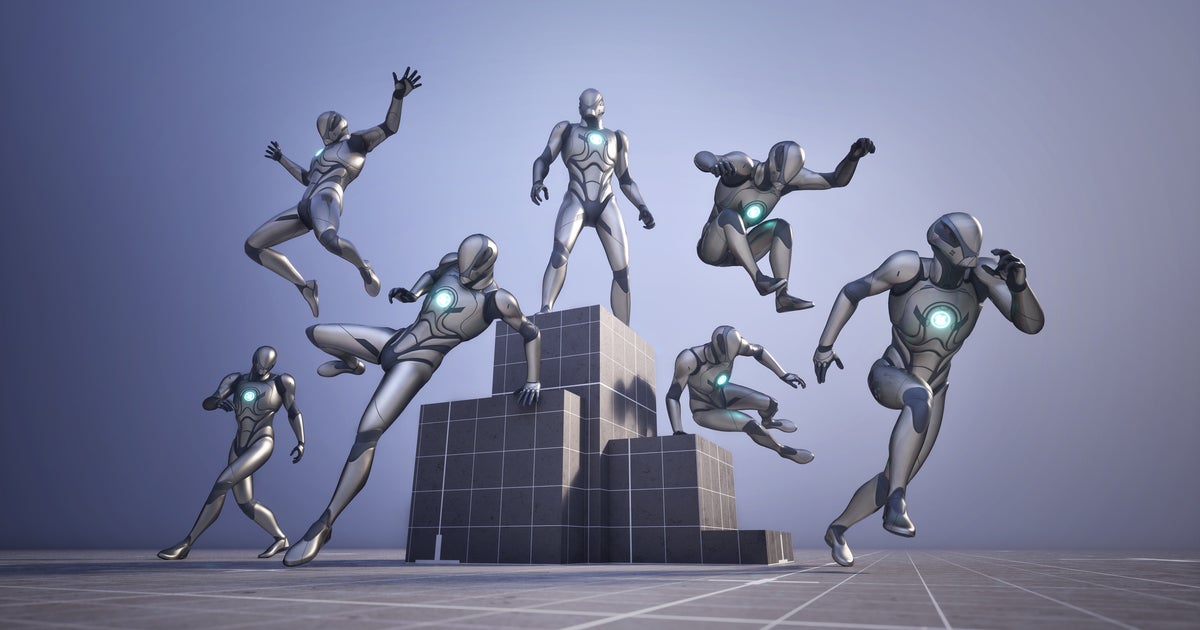The image appears to be a computer-generated graphic from a video game or futuristic scene, portraying seven men in steel suits resembling RoboCop. Each man is encased in a form-fitting robotic suit with helmets that conceal their faces, and a round light, akin to Iron Man's arc reactor, glows on their chests. The scene is predominantly gray with a bluish hue, creating a stark, metallic ambiance. The men are dynamically positioned around a series of three main cubes and a smaller step-like block, featuring a grid pattern. The men are depicted in various active poses: one is captured mid-run off the screen to the right, another leaps prominently into the air, while others are either jumping, standing with a hand on the block, or maintaining a poised stance, casting shadows that indicate an unseen distant light source. The arrangement of the blocks and the men suggests a sporting event or action sequence, accentuated by the high-energy movement and spatial depth.